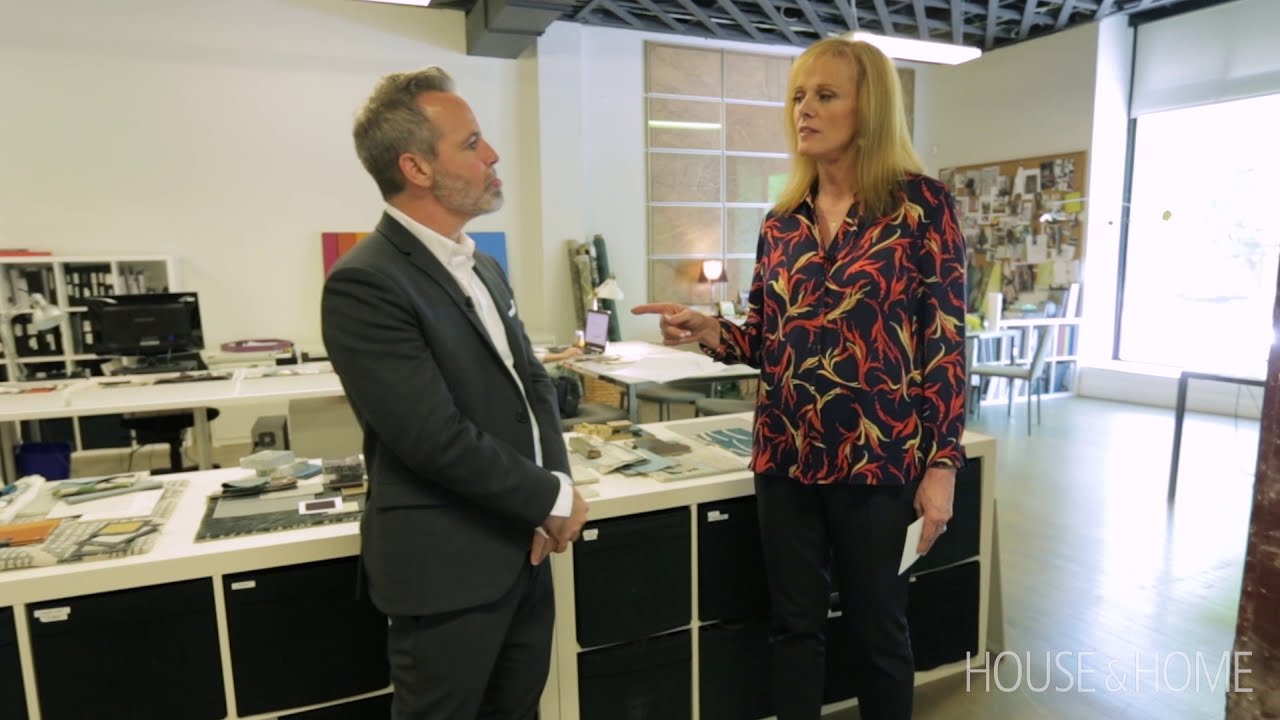In a brightly lit office adorned with large windows to the right, two individuals stand at its center on a hardwood floor, the words "House and Home" displayed in white letters in the lower right corner. The man, slightly shorter, is dressed in a gray suit with a white collared shirt, has short grayish-black hair, and sports a matching beard. He stands with his arms clasped at hip level, right hand over his left wrist, turning his profile slightly towards the woman. The woman, taller with shoulder-length mousy blonde hair, wears black trousers and a striking long-sleeved shirt with red and yellow flame patterns. She stands directly opposite the man, her right hand outstretched, pointing at him, while holding a white envelope in her left hand. The room exudes a creative atmosphere with a cork board pinned with various papers, visible computer monitor atop a white countertop, and a second countertop cluttered with papers and pictures, its base featuring black storage spaces.